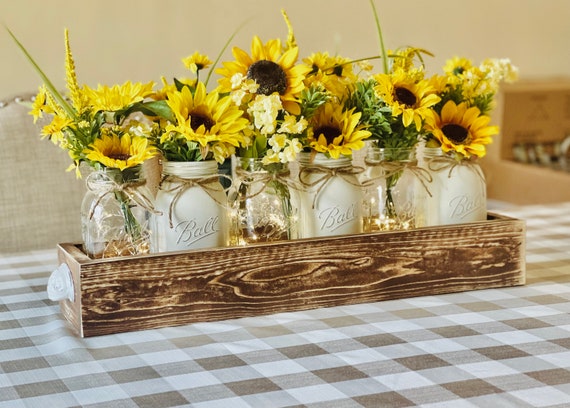This photo features a charming table decoration set on a brown and white checkered tablecloth. Central to the arrangement is a long, skinny rectangular wooden box with white handles on each side. The box holds six Ball mason jars, alternating between clear jars with tiny fairy lights and white jars. Each jar is adorned with a piece of burlap string tied into a bow around the neck. The jars are filled with artificial floral arrangements, comprising vibrant yellow sunflowers, goldenrod, small white and yellow flowers, and accompanying greenery. The enchanting display adds a rustic yet elegant touch to the setting. In the background, there's another surface, possibly a counter or a sink, visible but out of focus, providing depth to the scene.